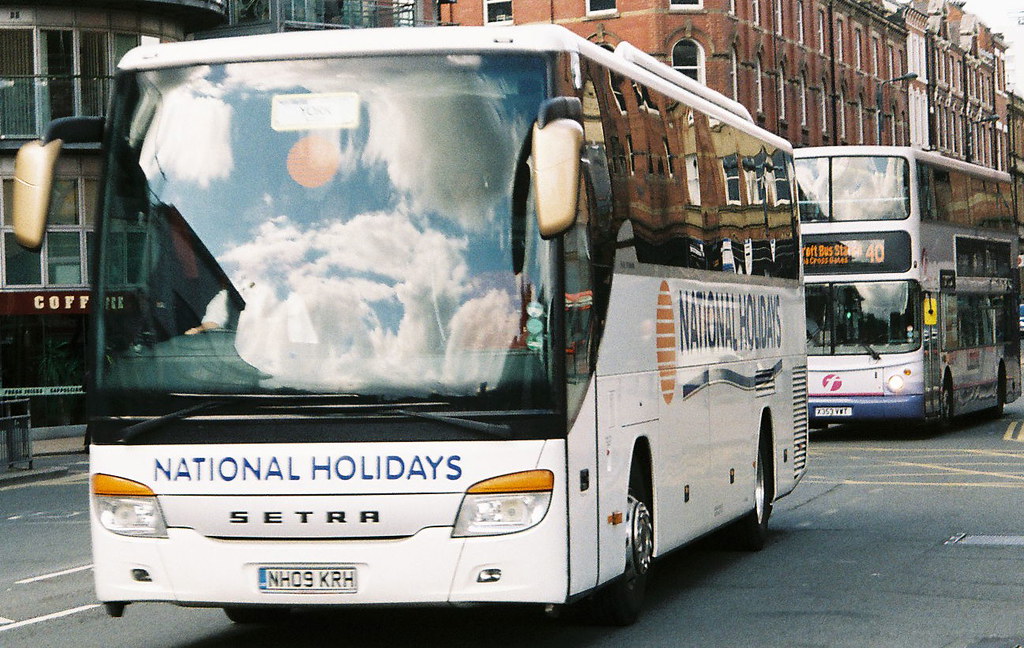This detailed photograph captures a bustling urban street in a downtown area, most likely in Great Britain, given the European-style license plates and English text. In the center of the image, two buses are prominently featured. The lead bus, a white excursion-style bus adorned with blue and orange markings, belongs to the "National Holidays" company, indicated by the text on its front. This bus has a license plate reading NH09 KRH and sports the SETRA brand logo. Behind it, a modern double-decker bus from a different company is visible. Both vehicles are driving along a standard asphalt road marked with paint, amidst an outdoor, mid-day setting.

To the left of the buses, there are multi-story brick buildings characteristic of an urban environment. Among them is a notable three-story building with ornate windows, featuring arch-topped designs, adding a historical charm to the scene. Additionally, a coffee shop occupies the ground floor of one of these buildings. The image's color palette includes shades of gray, yellow, white, orange, light blue, black, and brown, complementing the overall cityscape.